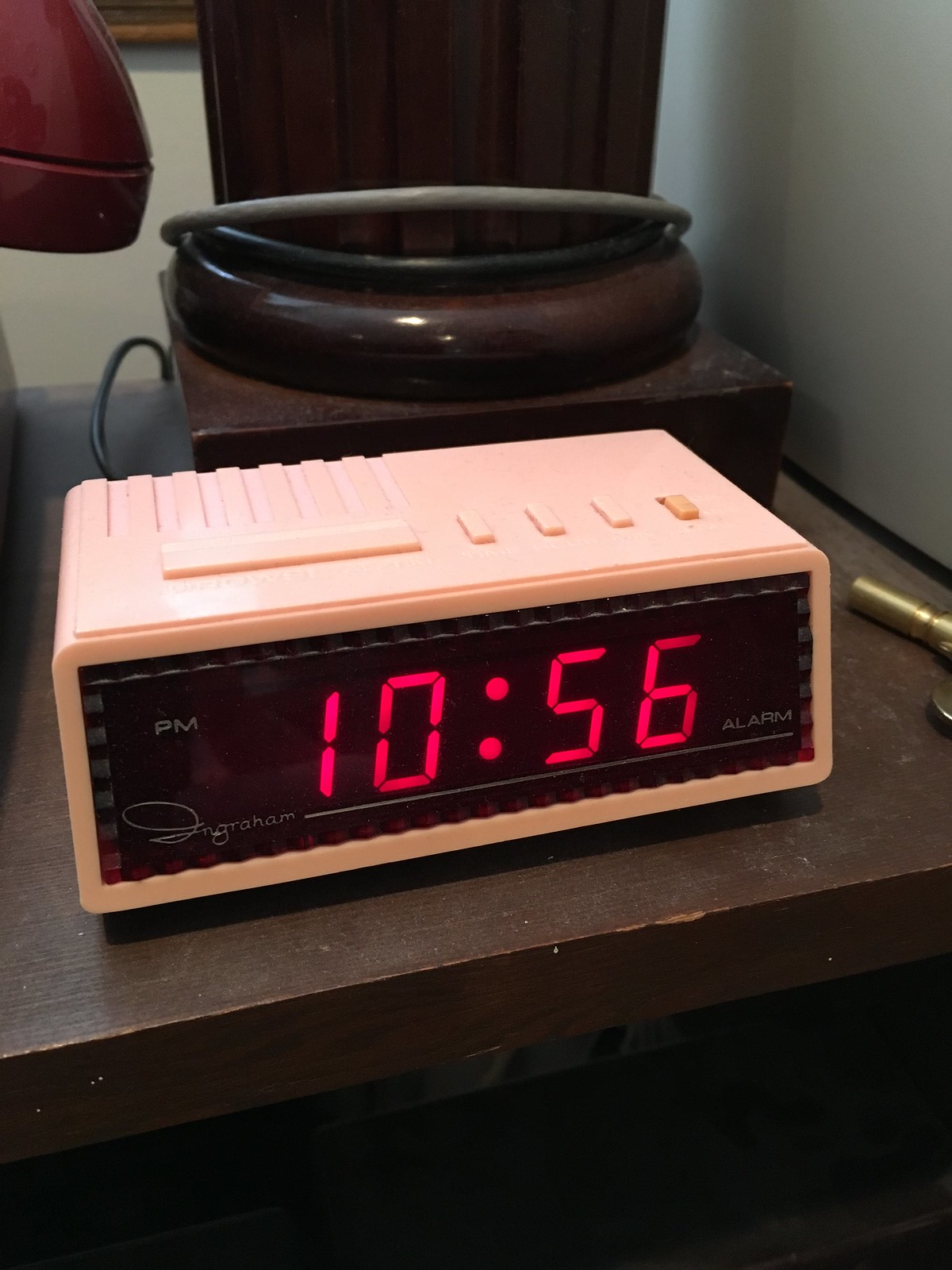This photograph, taken in portrait mode from the perspective of someone lying in bed, depicts a detailed and meticulously arranged nightstand scene. The focal point of the image is a digital alarm clock with a calming coral peach housing, which prominently displays the time "10:56" in bright red digits on its LCD screen with a black background. There are four small rectangular buttons and a long rectangular snooze button on its top, one of which is a hot pink color used for activating and deactivating the alarm. Inscribed on the screen are the indicators "PM" on the left and "alarm" on the right, along with the brand name "Ngram" and a signature. The clock sits atop a dark chocolate brown wooden nightstand, which shows signs of age with some dust and chipping.

Directly behind the clock stands the base of a large lamp, which has a dark chocolate brown, polished cylindrical shape with engraved lines and a flat, circular bottom. The lamp cord, partially gray and partially black, hints at a repair. To the right of the clock, a brass cylindrical object is visible but partially cut off, and a round piece of black metal accompanies it. On the left side, a vintage telephone with a red earpiece peeks into the frame.

The nightstand is set against a light gray wall adorned with the subtle outline of a light brown picture frame. The overall composition captures an intimate, indoor setting, emphasizing the stillness and functionality of a bedside environment.